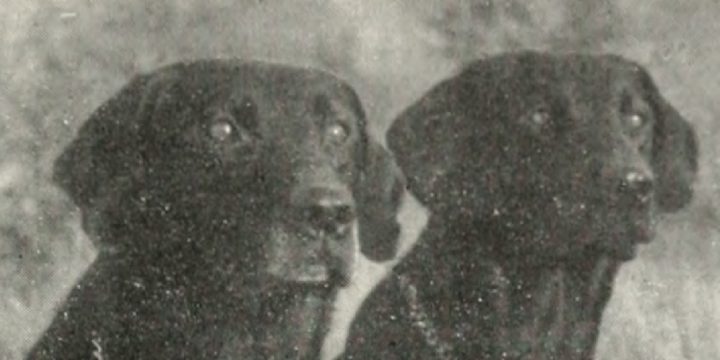The black and white image captures a close-up of two dogs, possibly Labradors or Dachshunds, sitting side by side. Only their heads, necks, and part of their shoulders are visible. Both dogs share similar features, including long, floppy ears, glossy dark eyes, and shiny black noses. Although their exact breed is uncertain, they look remarkably alike, with one dog appearing slightly larger than the other. They are gazing intently at something just to their left, with neither appearing particularly happy. The background is an indistinct blur of varying shades of gray, black, and white, giving the impression of an old, possibly snow-dusted, scene. The entire image is grainy and dotted with white spots, suggesting it might be an aged photograph or a scanned newspaper clipping. This detailed and somewhat pixelated portrayal highlights the calm and composed demeanor of the dogs.